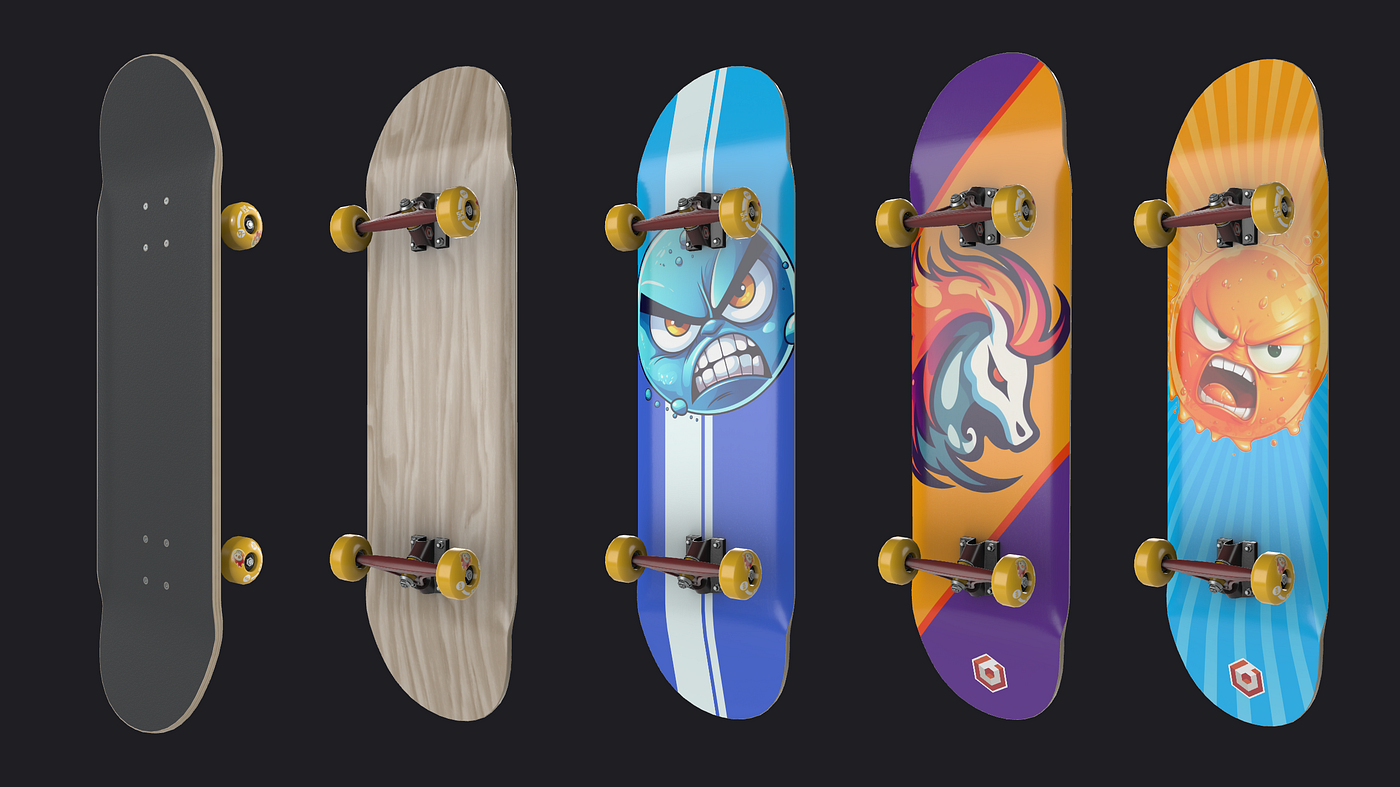This digital image showcases five distinct skateboards, set against a black background, each illustrating unique features in what appears to be 3D renderings. The skateboard on the far left displays its black grip tape on the top side and yellow wheels, highlighted by its tan color and secured by four metal screws on each end of the trucks. The second skateboard from the left reveals the bottom side, showing a darker wood grain with red trucks and yellow wheels, with no additional design details. The central skateboard features a striking blue gradient design that transitions from light blue at the top to a royal blue at the bottom. This board is marked by a white stripe running vertically down the left side and boasts an angry blue face with gritted teeth, yellow-orange irises, and furrowed brows. The fourth skateboard depicts a vibrant image reminiscent of a school mascot, with a white horse sporting a fiery red and yellow mane, a diagonal orange stripe, and top and bottom sections in purple. Finally, the skateboard on the far right presents another angry emoticon, this time a yellow face with raised eyebrows and an open-mouthed expression. This board features a two-tone color scheme with a yellow upper half and blue lower half, accented by radiating lines that are a slightly darker shade than their respective backgrounds.